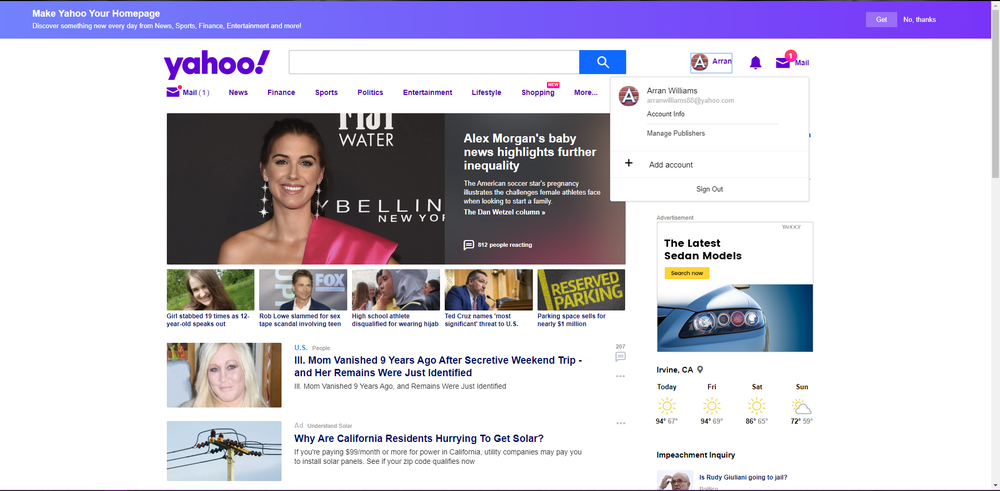The image shows Yahoo's homepage with notable elements organized across the layout. 

In the top-left corner, the familiar purple Yahoo logo is prominently displayed. At the top, there's a search bar accompanied by a blue search button. On the right side of the page, a user's avatar is visible, featuring a brown background with a white "A" inside it, indicating an active login session. Someone appears to be clicking on this avatar, causing a white pop-up box to appear with the name "R. Amon Williams," although it's blurry and hard to read. An email address is shown beneath the name, alongside menu options like Account Info, Manage Publishers, Add Account, and Sign Out.

Flanking the avatar are two icons—a purple notification bell and an envelope labeled "Mail" with a red circle containing a white "1," indicating a new message. Below the search bar, a horizontal menu showcases links to sections like Mail, News (in purple), Finance, Sports, Politics, Entertainment, Lifestyle, Shopping, and more.

The central section of the page features a large rectangular box highlighting the top news story with a picture of Alex Morgan wearing a pink dress. The headline reads "Alex Morgan's baby news highlights further inequality," set against a gray background with white text. 

Beneath the main story are five smaller news stories with images:
1. A girl with brown hair.
2. Actor Rob Lowe.
3. A woman wearing a head covering.
4. Ted Cruz.
5. A reserved parking sign with big yellow letters.

Under these, additional articles are listed:
- On the left: An article with a blonde woman's picture and a headline in blue, "Illinois ill mom vanished nine years ago after secretive weekend trip – her remains were just identified," followed by small gray text.
- Below it: An article featuring a power line image with the headline, "Why are California residents hurrying to get solar?" followed by gray text.

On the right side:
- A panel section advertises the latest sedan model, featuring a white headlight picture, followed by a weather widget showing forecasts for Irvine, CA, with icons and temperatures, though the numbers are blurry.
- Continuing below, there's an article on the impeachment inquiry, with a picture of an older man and a headline asking, "Is Rudy Giuliani going to jail?"

This detailed breakdown captures the intricate details of Yahoo's homepage, from key navigation elements to the variety of news stories presented.